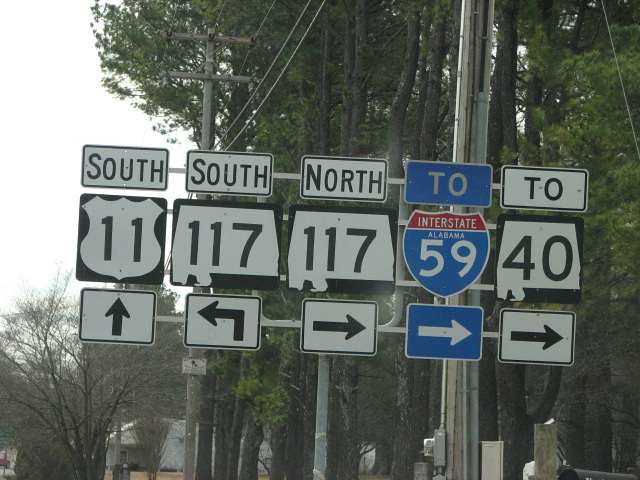This image is a close-up shot of five roadway signs meticulously aligned side by side, each directing travelers to different routes. From left to right, the signs read: "South Route 11," distinguished by its simple white number 11 on a black background with a route symbol. Next is "South Route 117," followed by "North Route 117," both similar in style. The fourth sign stands out as an Interstate sign, adorned in blue and reading "Interstate Alabama 59." The final sign in the series displays a white number 40 on a black background, with the word "To" above it, indicating a directional guide to Route 40. The arrangement provides clear pathways for navigating various routes and interstate directions.